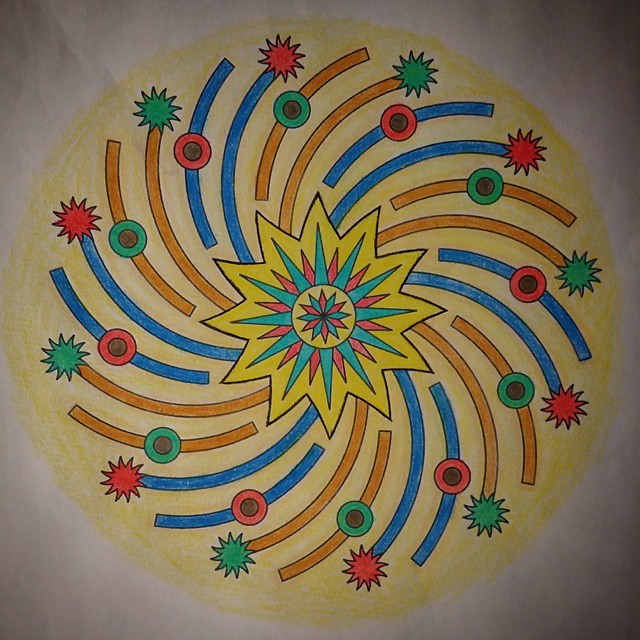A meticulously colored-in image on a white sheet of paper reveals an intricate design centered around a vibrant yellow star. This star, which sits at the heart of the composition, contains a smaller multi-pointed pink star intertwined with a teal star adorned with radial spikes. Inside the teal star is a circle featuring a flower-like pattern reminiscent of a poinsettia, with alternating green and pink leaves. 

Surrounding the central star is a larger star outlined with additional points extending outward, forming a medallion-like structure. From the vertices of the star, numerous curved lines spiral outwards in a pinwheel fashion, filled in with alternating blue and orange hues. Each pair of these lines is decorated at the tips with either double circles or star shapes, adding to the layered complexity of the design. The blue lines feature orange stars, while the orange lines have teal stars, seamlessly blending the colors together.

Overall, the image uses a harmonious palette of blues, oranges, greens, pinks, and yellows, suggesting it may have been skillfully colored with crayons or colored pencils, evoking a sense of both childlike wonder and artistic precision.